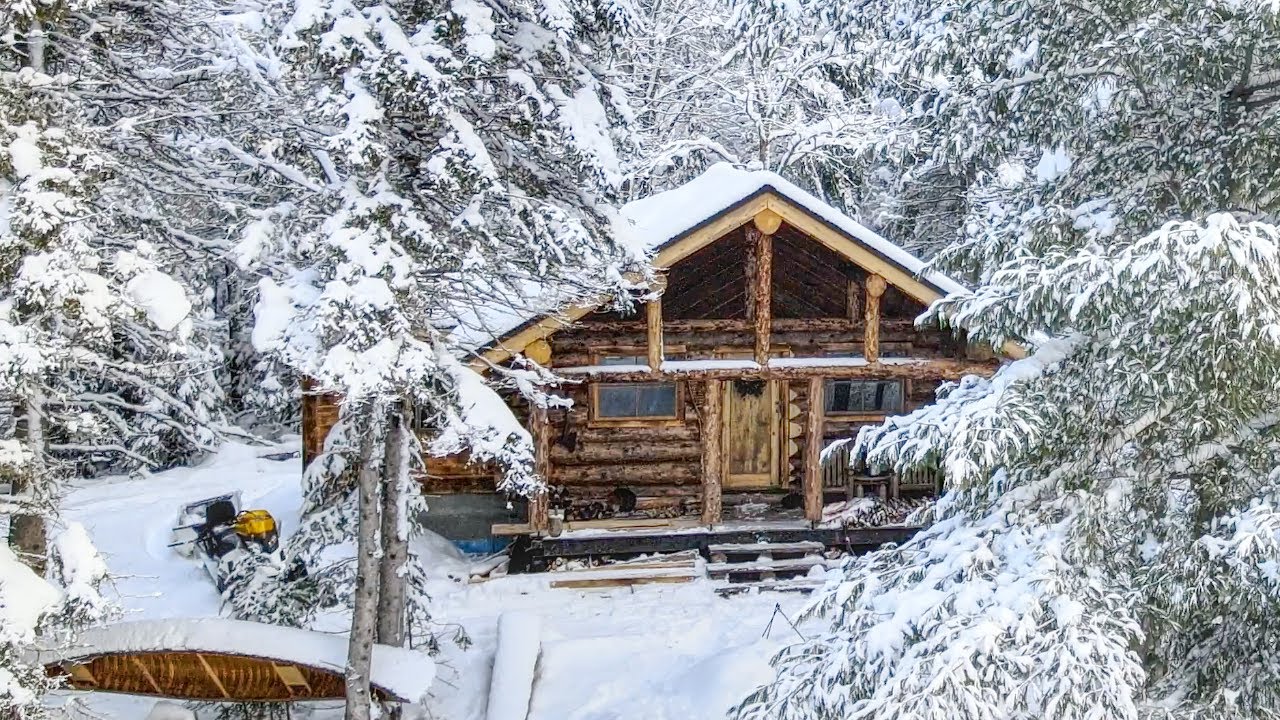In this picturesque winter landscape, a secluded log cabin stands amidst a dense covering of snow. The scene is surrounded by tall green trees, their branches heavily blanketed in thick, pristine snow, resembling a Christmas card illustration. At the center of the image, the cabin boasts a high triangular roof and sturdy, dark brown timber walls. Fronted by a small set of wooden steps laden with snow, the cabin features a lighter wooden door and two windows that face out onto the tranquil, snowy scene.

To the left of the cabin, various pieces of equipment are visible. A canoe, turned over on its side to prevent it from filling with snow, is strategically mounted between two trees in the lower left-hand corner. Near the canoe, there appears to be an overturned grill and possibly a snowmobile, evidence of human activity in this otherwise serene setting. The entire area exudes a sense of quiet solitude, with the untouched snow adding to the enchanting, wintry atmosphere.